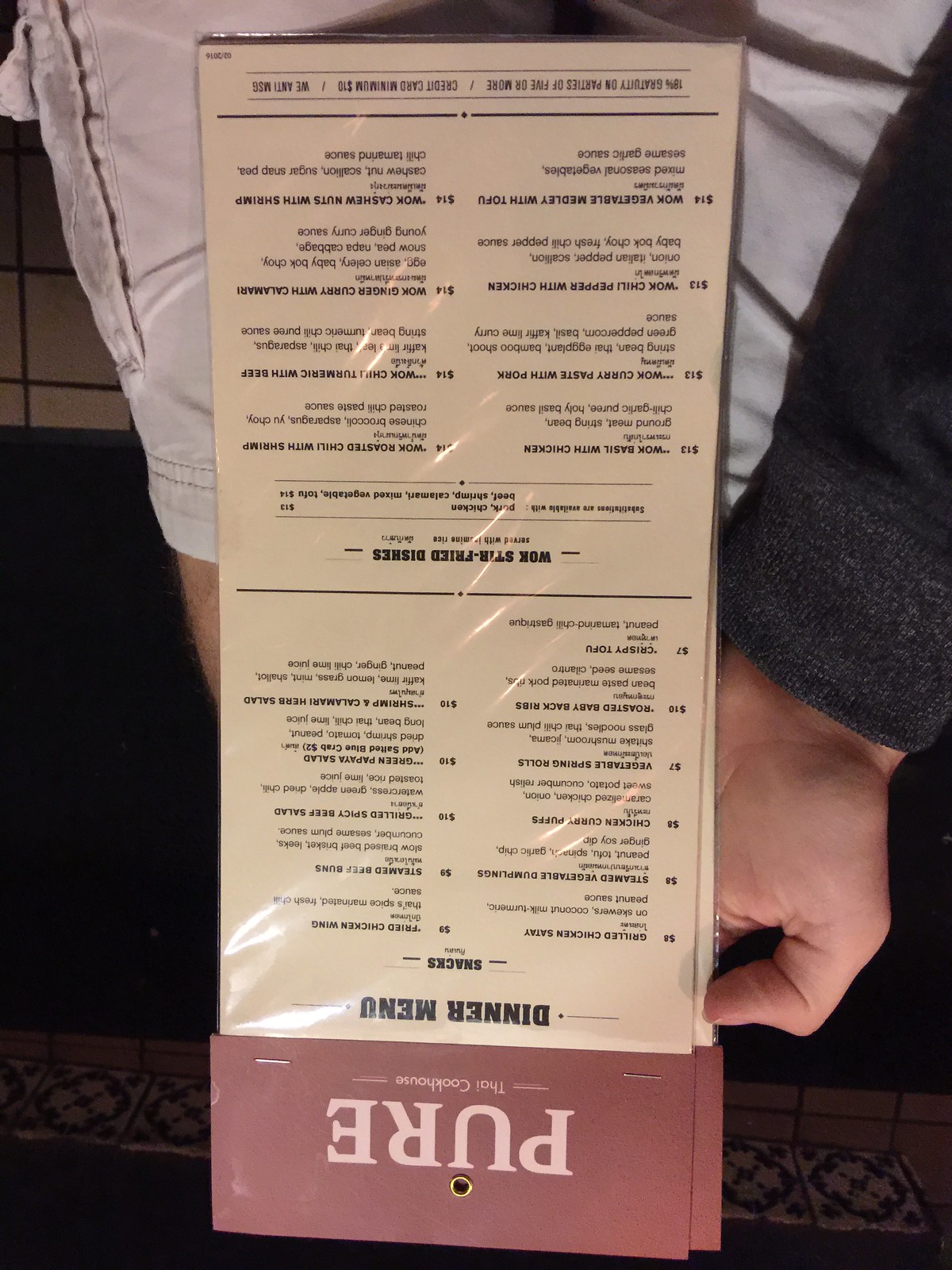Here is a refined and detailed caption for the given image:

---

The image is an upside-down, landscape-oriented photograph of two identical packets. The packets feature a maroon-colored top section with light pink lettering that reads "P-U-R-A The Cookhouse." Each packet has gold eyelet circles at the top, making them suitable for hanging on a wall. The edges of the packets are stapled, and a plastic cover encloses the contents. 

Through the plastic cover, the dinner menu is visible, printed in black text. The menu is organized into two columns. The first column lists:

- Snacks: Grilled chicken, steamed vegetable dumplings, chicken curry, vegetable spring rolls, roasted baby back ribs, crispy tofu

The second column includes:

- Fried chicken wings, steamed (illegible), grilled spicy beef, green papaya salad, shrimp and calamari herb salad 

Between the two columns is a prominent black stripe. Below this, another section titled "Wok Stir-Fried Dishes" begins. The first column in this section lists:

- Wok basil with chicken
- Wok curry paste with pork
- Wok chili pepper with chicken
- Wok vegetable medley with tofu

The second column lists:

- Wok roasted chili with shrimp
- Wok chili turmeric with beef
- Wok ginger curry with calamari
- Wok cashew nuts with shrimp

Despite the image being upside down, these elements combine to provide a clear view of the packet's design and menu details.